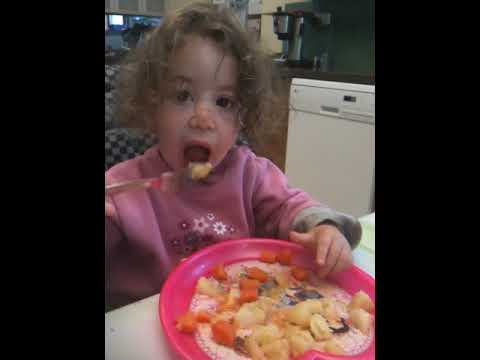A photograph captures an indoor setting, possibly a kitchen or living room, featuring a young toddler, around two to three years old, with long brown hair. The child, whose gender is ambiguous, is seated in a black and grey checkered chair at a white table. She is wearing a pink and gray sweatshirt adorned with little daisy flowers and appears to be in her pajamas, hinting that it might be morning. In her right hand, she clutches a pink fork, which she uses to dig into a large, heart-shaped pink plate filled with colorful food items, including what appears to be potatoes, carrots, and rice. A piece of potato is held in her left hand. The background includes a shelf with a metal kettle and a window, while the presence of large black rectangles framing each side of the photo adds to the overall composition. The image is devoid of any text.